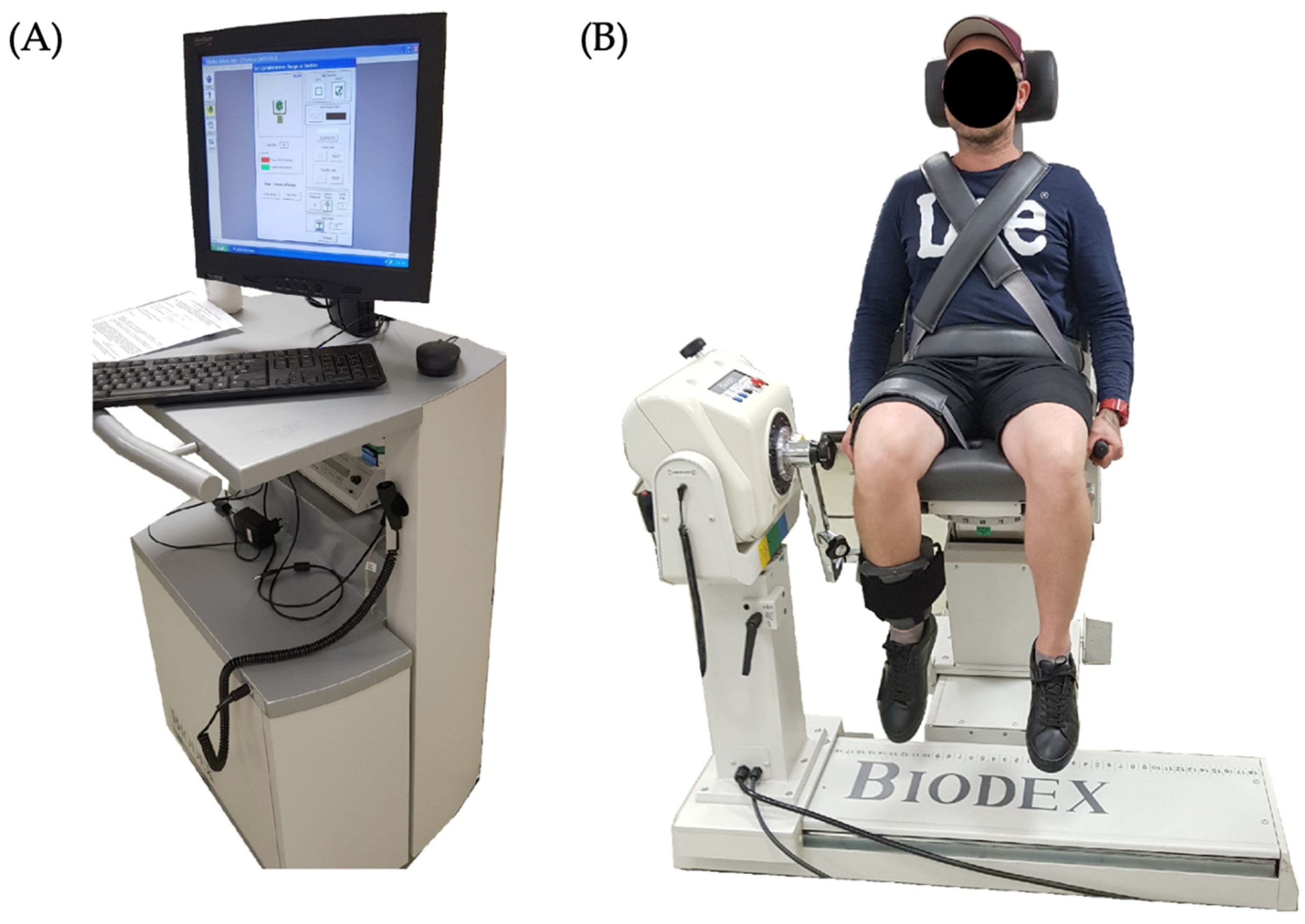The photograph depicts a medical device setup used for physical rehabilitation. On the left, labeled 'A,' is a computer workstation featuring a black keyboard and mouse on a beige shelf, connected to a PC screen displaying a chart, although the details are indistinct. The computer, adorned with various cables, appears to monitor or control the operations of the adjacent equipment.

On the right side, labeled 'B,' a man is seated in a Biodex medical device, primarily cream and gray in color, resembling the base of a treadmill but without a running track. The man, whose face is obscured by a privacy circle, wears a red baseball cap, a blue long-sleeve T-shirt with partial "LEE" branding, and black shorts. He is secured to the gray leather chair by an array of straps across his chest, midsection, and right thigh, with a rigid plastic brace attached to his right ankle, connected to a rotary mechanism – presumably for leg rehabilitation exercises. His left leg hangs freely, and he grips a handle with his left hand. The setup includes numerous cables and control elements, suggesting a comprehensive system for monitoring and adjusting therapeutic activities. The base of the device prominently displays the brand name "Biodex."